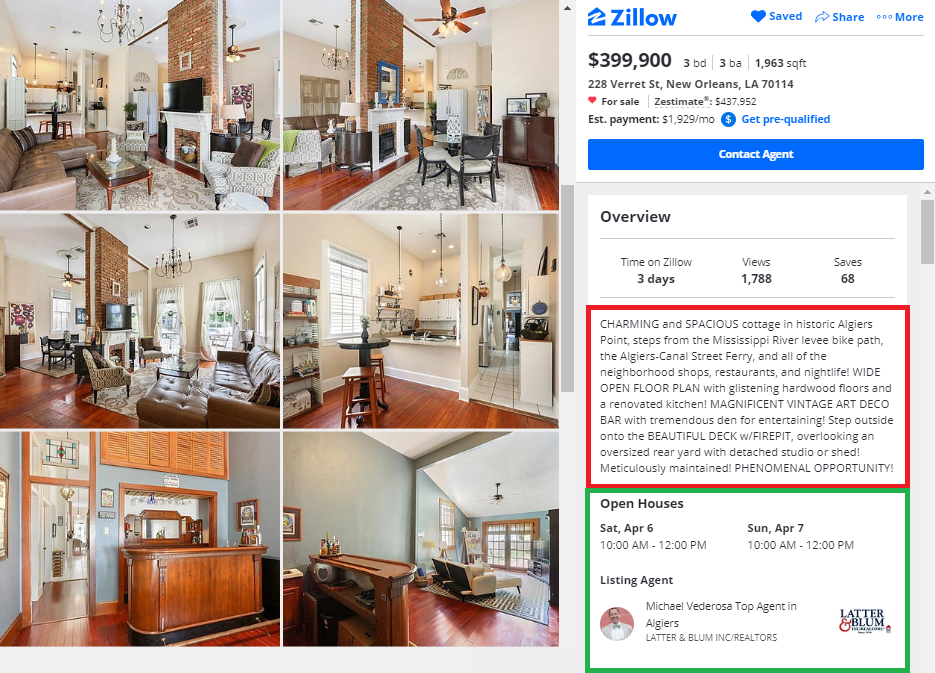This is a left-to-right horizontal image from Zillow, accessible on computers and smart devices. The background features a blend of gray tones and white areas, likely influenced by the computer screen. On the left-hand side, there are six smaller images arranged in a 2x3 grid, showcasing different rooms in the home. 

On the right-hand side, the Zillow logo appears in blue, next to a heart icon labeled "Save," a share button, and a "More" button. Below this, pertinent information about the property is presented in bold black text: the home is listed for $399,900, features three bedrooms, three bathrooms, and spans 1,963 square feet. The address is provided, indicating the home is for sale, along with the estimated monthly payment, a "Get Pre-Qualified" button, and a "Contact Agent" button.

Further details include an overview section with the home's time on Zillow (three days), the number of views (1,788), and total saves (68), all outlined in red. The open house schedule and listing agent details are highlighted in green. Additional information can be accessed via a scroll bar on the right.